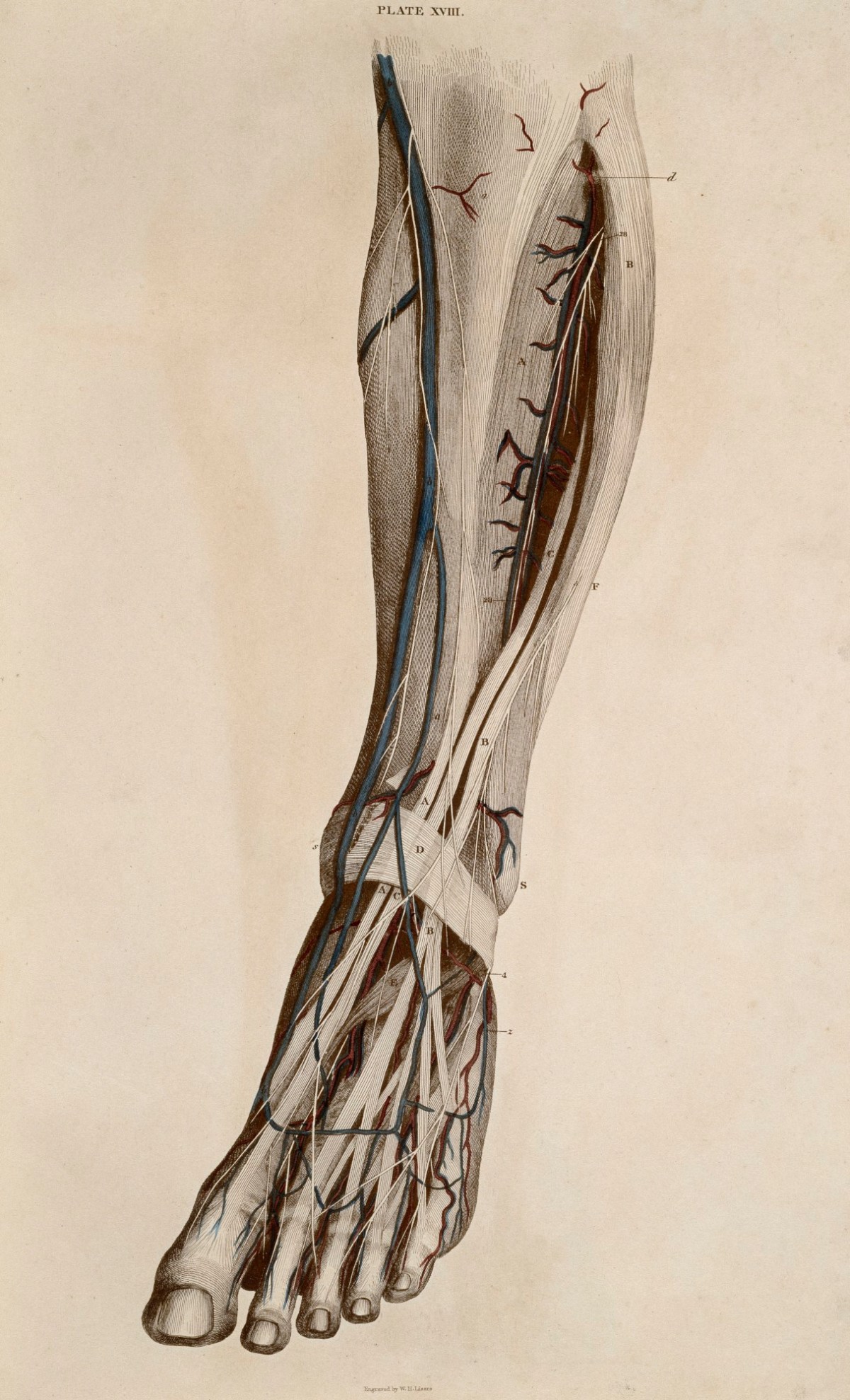This is a vertically aligned rectangular image, an intricate pen and ink drawing that appears to be from an anatomical book or a slide for an anatomy class. The paper has a weathered, light brown color with a yellowed appearance. At the very top, small printed words read “Plate NV...” followed by an unclear letter. 

The drawing depicts the lower part of a human leg, from just below the knee to the foot. Detailed anatomical features are meticulously illustrated. The skin is either transparent or pulled away, revealing internal structures. On the left side, blue-colored arteries run from the shin down to the toes, branching out vividly. Dark brown and red are used to indicate blood vessels and muscles, with intricate branches and details.

The image showcases the bones with great precision, extending from the shin, past the ankle, and into the toes. Toenails are visible on each toe, enhancing the realism. Around the ankle, a white band, resembling a piece of tape or ligament, wraps snugly. Additionally, the drawing contains labeled markings and arrows, likely pointing to a glossary or legend that explains each anatomical part.

This highly detailed, educational illustration provides a comprehensive view of the lower leg and foot, combining artistic skill with scientific accuracy.